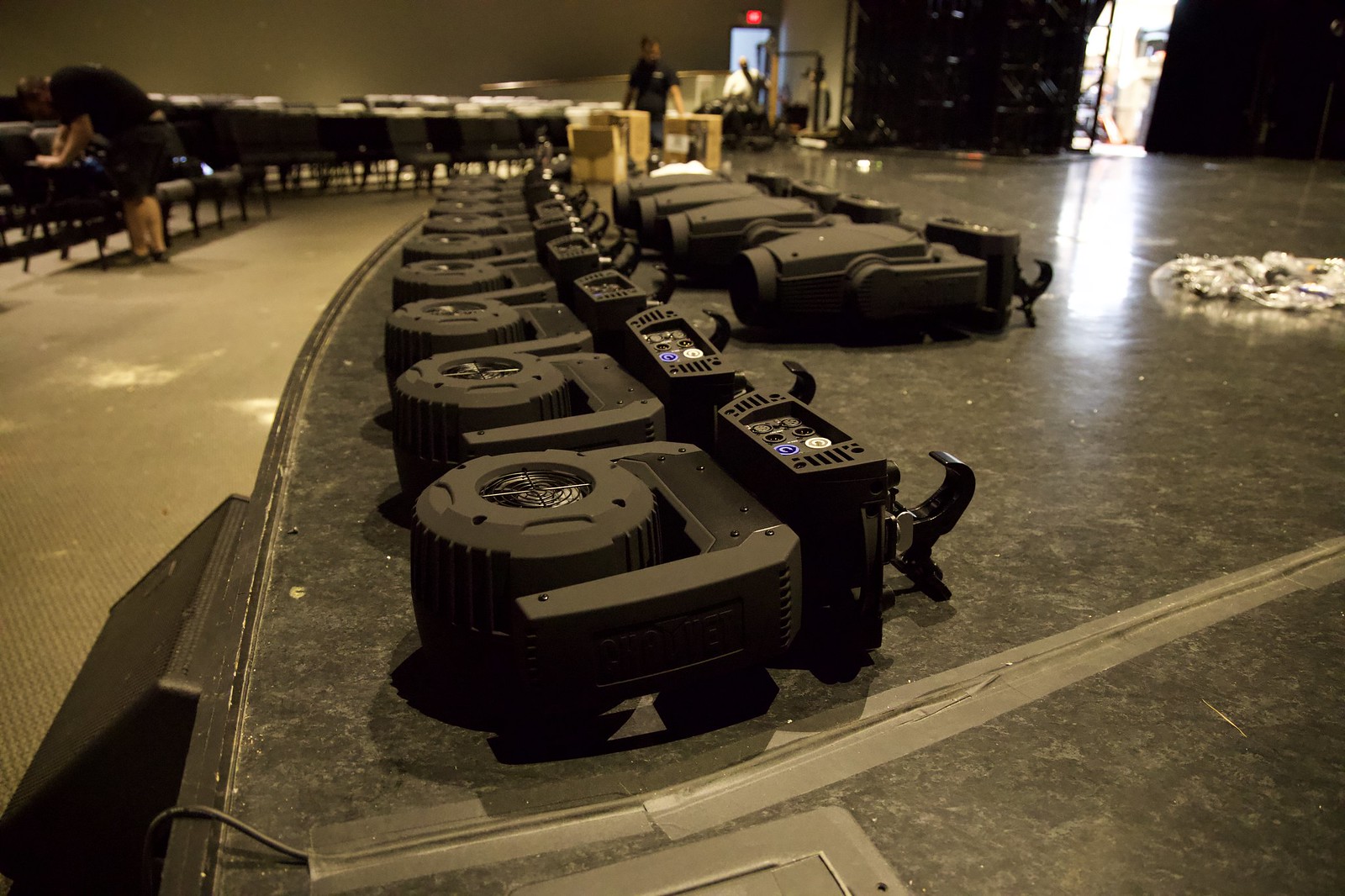This indoor color photograph captures a detailed view of a stage setup, featuring a long row of stage lights used in lighting decorative optics for performances. The row begins in the foreground and extends towards the background, with approximately 10 moving head LED lamps visible. These lamps are equipped with bar hanging grips for mounting on bars or framework. To the right, there are larger LED heads with motorized mounts, capable of producing beams of colored light, optics, and strobe effects through fog machines. The stage surface is covered in a plasticky material, marred with brown splotches, and duct tape secures wires running towards the lights. The stage curves slightly up into the background on the right, where we can see an opened black curtain with light filtering through. In the upper left, seating for the auditorium is visible, with chairs and people working, possibly prepping for a concert or taking down equipment afterward. A person in shorts and a black shirt leans over on the left, engaged in the setup process. The overall scene presents a snapshot of the meticulous preparation involved in stage lighting for live performances.